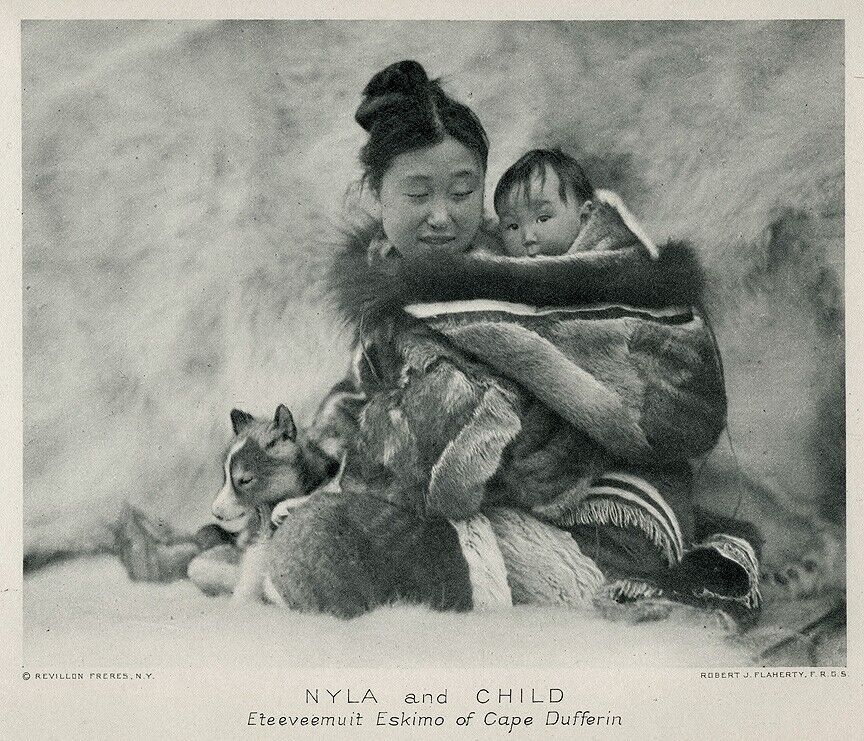The faded, antique-style black and white photograph depicts a serene moment between a mother of Eskimo descent and her child. The mother, Nyla, is seated cross-legged and wrapped in a luxurious fur coat that envelops both her and her baby, who peeks out from the hood with wide-open eyes. Her long black hair is tied back into a bun, and she gazes lovingly towards her child. Nestled in her lap is a small puppy with a white stripe on its face and black stubby ears, also wrapped in fur. They are seated on an expansive animal rug, with more fur lining the wall in the background. The bottom left of the photo features the slightly obscured shape of an animal, possibly a cat or fox, with closed eyes. The photograph is credited to Robert J. Flaherty, FRGS, and a copyright by Revlon Paris, New York. The text at the bottom reads, "Nyla and Child, Etivemuit Eskimo of Cape Dufferin."